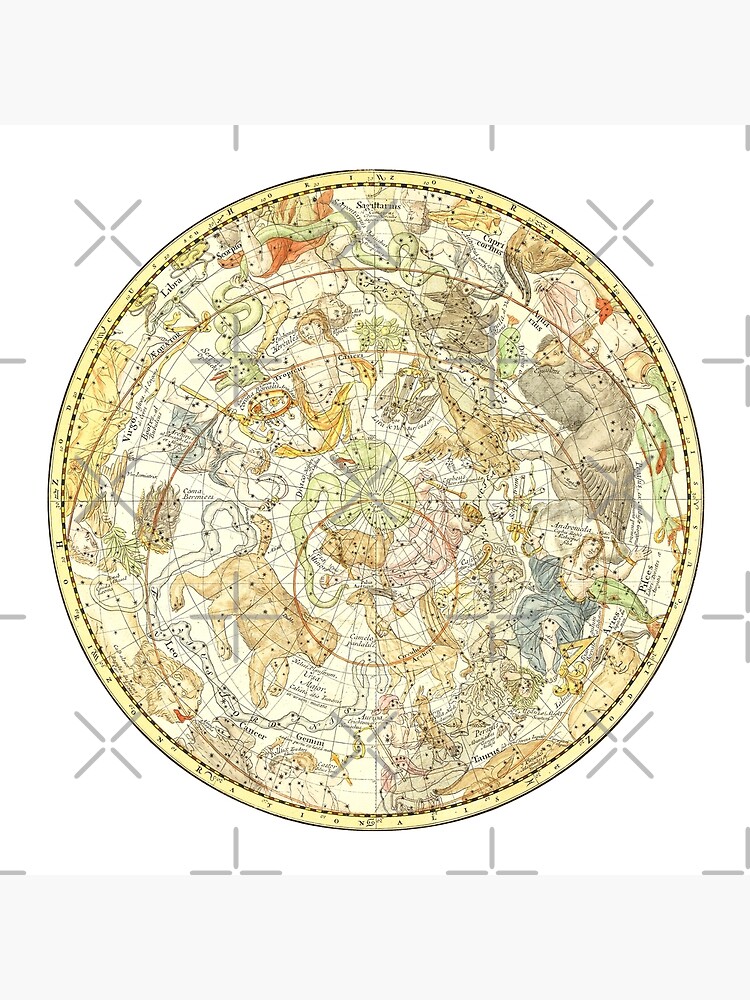The image is a detailed circular illustration, resembling a sky atlas or a globe, densely populated with a variety of intricately painted animals and mythological figures. Encompassing the focal point, the outer rim features several astrological signs and measurement markings, all rendered in fine detail. Inside the circle, the illustrations include a diverse array of creatures such as dogs, leopards, gazelles, snakes, goats, and bears. Prominent among these is a topless woman adorned in a blue robe near the bottom-right, and a man draped in gold fabric, reminiscent of a Greek god, centrally located with a snake coiled around him. The constellations, though faint and interspersed with star-like dots, include representations of Leo, Gemini, and other zodiac signs. Splashes of orange, yellow, and light green colors dominate the color scheme, with additional touches of red in the woman's hair and her drape. Gray X's are subtly visible around the perimeter of the photograph.